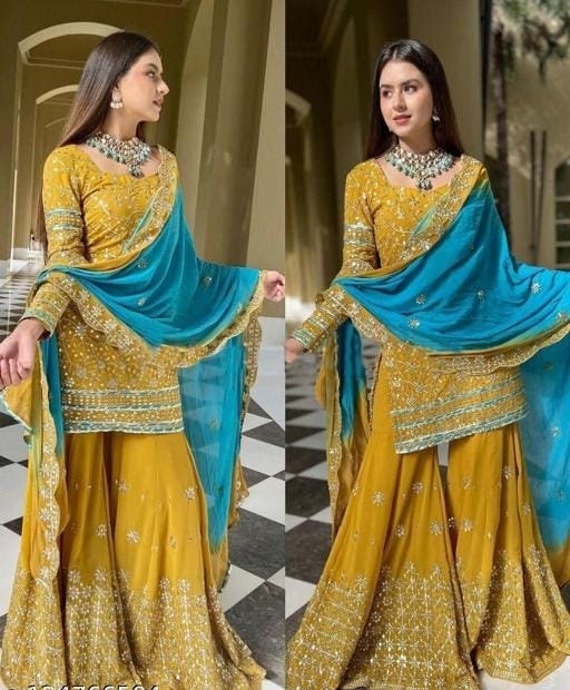This image features the same young woman in two panels, each showcasing her from different angles. She appears to be in her early 20s and has long brown hair. The setting includes a distinctive black and white checkered floor, a gold door with a white arch, and a gold curtain visible in the left panel. The woman is adorned with an ornate, multi-strand beaded necklace and matching earrings. She dons a vibrant, long yellow gown with a floral pattern that extends from her shoulders to beneath her ankles. Her attire also includes an overlaid, semi-transparent turquoise blue shawl, which she holds between her outstretched arms. Both panels capture her in the same outfit, emphasizing the elegance of her clothing and accessories as she gazes in opposite directions in each image.